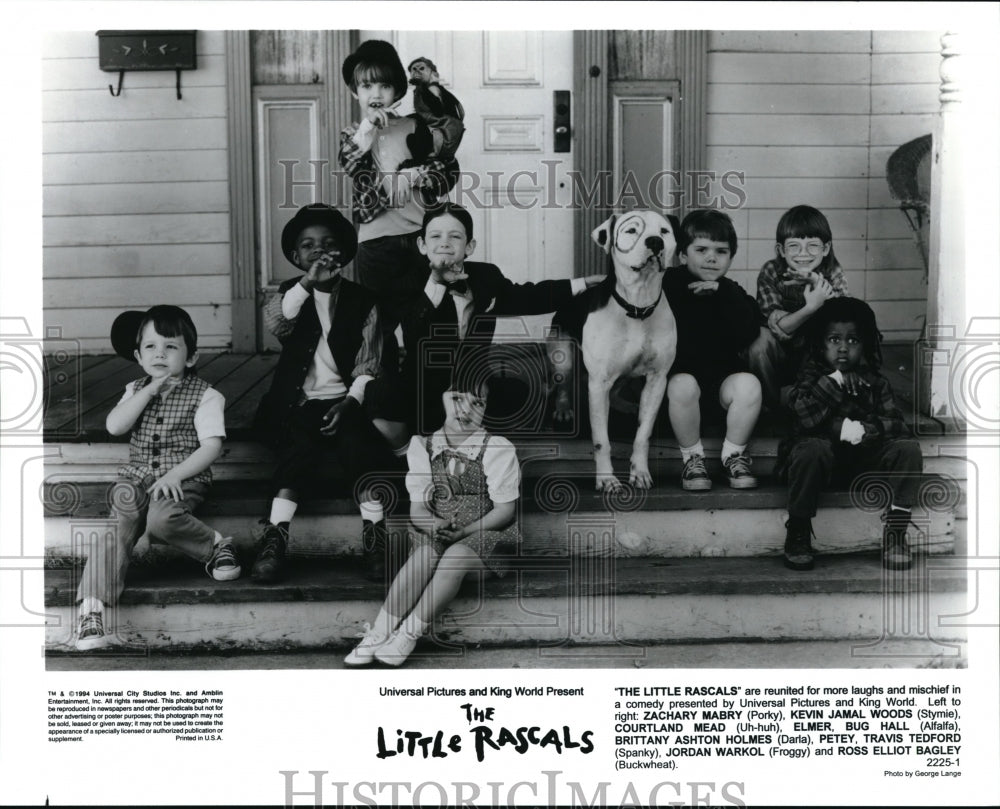This detailed vintage promotional photograph of "The Little Rascals" is sourced from Historic Images, as indicated by the watermark imposed in the upper middle part. The black-and-white image captures eight children dressed in the iconic attire familiar from the classic show, posing on the steps of a home with a visible mailbox to the left of the door. Among the recognizable characters are Alfalfa, identifiable by his signature hairstyle, and Buckwheat, along with Darla, who sits with her hands folded on her lap. A boy stands at the top of the stairs holding a monkey in his left hand and wears a small derby hat. Central in the group is a mostly white dog with a distinctive black ring around its right eye, likely named Spot. Most of the children are engaging in playful antics, with several holding their fingers extended in front of their chins, adding to the whimsical nature of the scene. The photograph features both black and white children, highlighting the diverse cast from the show. The bottom of the image reads "The Little Rascals" in black text, with additional, unreadable text to the side, and it evokes a sense of nostalgia for the original movie or series.